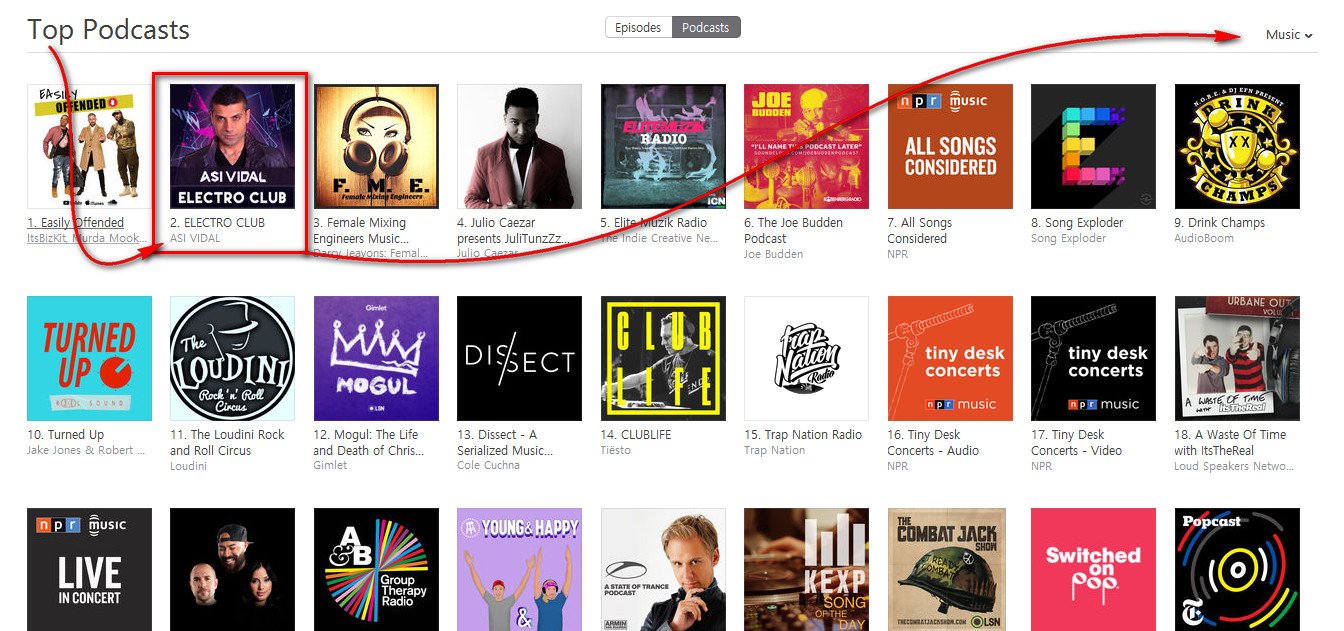Displayed is the interface of a digital audio platform, showcasing an array of podcasts and music selections. The top-left corner prominently features a label, "Top Podcasts," with tabs delineating between podcasts and their episodes. The current selection toggles between "Podcasts" and "Music," indicated by a visible dropdown box offering further category options.

Beneath this header, a series of three rows are populated with album artworks, each row containing nine distinctly illustrated covers. A curvy arrow directs attention from the first album on the leftmost side, weaving down and then paralleling the row before finally pointing back up to the "Music" dropdown box.

Highlighted albums in the first row include titles such as "Easily Offended," "Electro Club," featuring a female DJ, followed by "Julia Caesar Elite Music," "The Joe Bud Podcast," "All Songs Considered," "Song Exploder," and "Drink Champs." 

The second row presents "Turned Up," "Uni Rock," "Mogul: The Life and Death of Chris Lighty," "Club Live," "Trap Nation Radio," "Tiny Desk Concerts (audio version)," "Tiny Desk Concerts (video version)," and "A Waste of Time."

Lastly, the third row offers more selections: "Live in Concert," another set of nine covers without direct descriptions. Among these, notable titles are "Young and Happy," "Gaba Jack," "Switched on Pop," each item displaying vibrant album artwork against a white background.